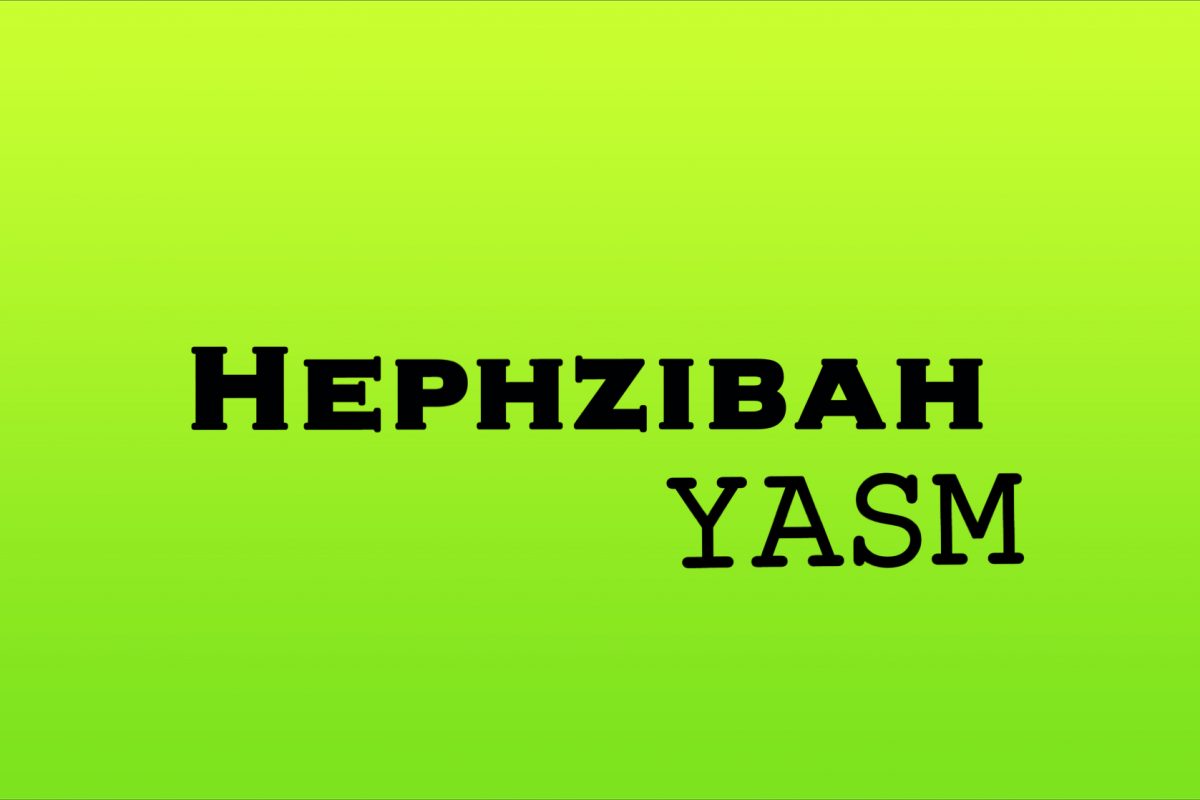The image features a neon lime green background with a slight gradient, transitioning from a more yellowish green at the top to a distinct lime green at the bottom. Prominently displayed in the center of the image in bold black capital letters is the name "HEPHZIBAH," with the first "H" slightly taller than the other letters. Directly below this, in a thinner typewriter-style black font, is the word "YASM," all in uppercase and right-aligned with the last letter of "HEPHZIBAH." The overall design is horizontally oriented, with the text forming a rectangular shape within the green background.